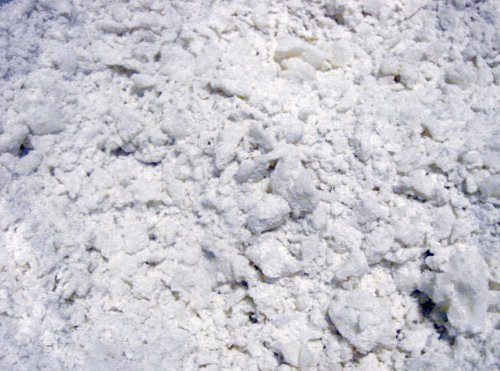The image depicts a textured, rocky surface scattered with white chunks, possibly resembling snow, cottage cheese, rock salt, or insulation material. The chunks vary in size, with larger, more prominent rocks concentrated in the center and bottom right, while the top left and bottom left areas appear smoother and more uniform. Shadows cast beneath the chunks create a play of light and dark, adding black hues that suggest depth. The coloration shifts from white and cream to almost purplish tints, especially towards the top, contributing to an overall bright yet varied appearance. The scene could either represent a rocky hillside or a flat surface viewed from above, making it challenging to determine the precise nature of the terrain.